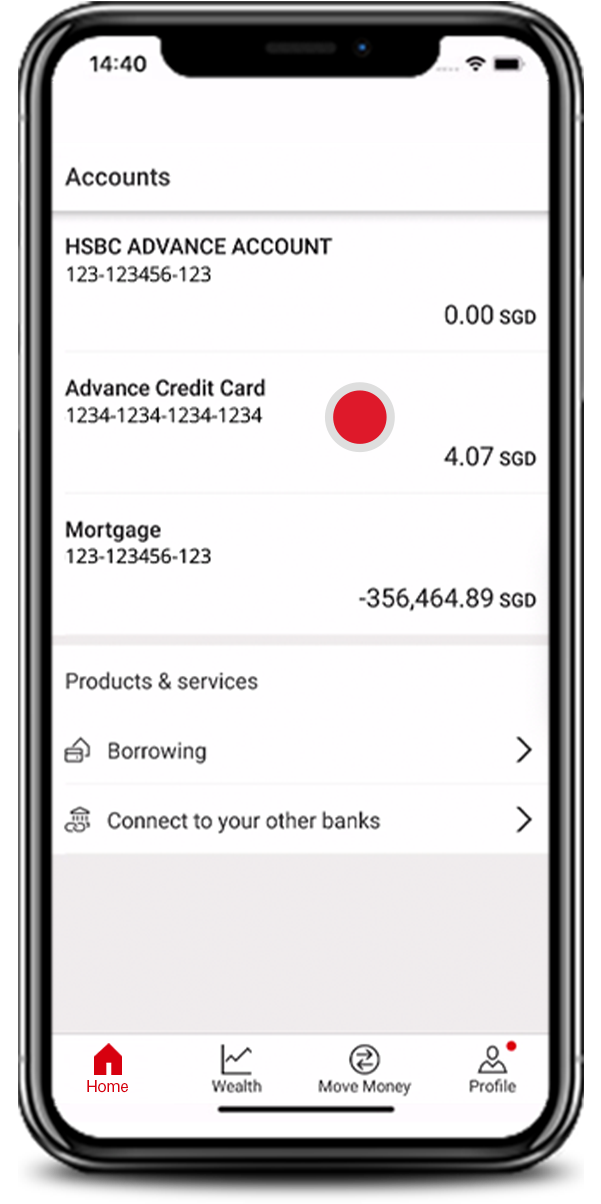This image is a detailed screenshot of a banking app displayed on a black-outlined cell phone. In the upper left-hand corner of the screen, the time is shown as 14:40, while the upper right-hand corner features a full Wi-Fi signal icon and a fully charged battery icon.

Underneath this, the section labeled "Accounts" is displayed in black text. Below this title, the first account listed is an "HSBC Advanced Account" accompanied by the account number: 123-123456-123. To its right, the balance is shown as 0.00 SGD. Beneath this, the next entry is "Advanced Credit Card" with the account number: 1234-1234-1234-1234. To its right, there's a red circle with a grey outline indicating the card status, and a balance of 4.07 SGD is shown.

Following this, the next entry is for a mortgage account with the account number 123-123456-123, which displays a substantial balance of 356,464.89 SGD to its right. Below the account listings is a section titled "Products and Services" in black text, followed by two options: "Borrowing" and "Connect to Your Other Banks," each with a right-pointing arrow next to them.

At the bottom of the screen, various navigation icons are arranged: a red home icon in the bottom left-hand corner, followed by a wealth icon represented by a line graph, a "Move Money" icon depicted as a circle with left and right arrows, and in the bottom right-hand corner, a profile icon with a red circle above it.